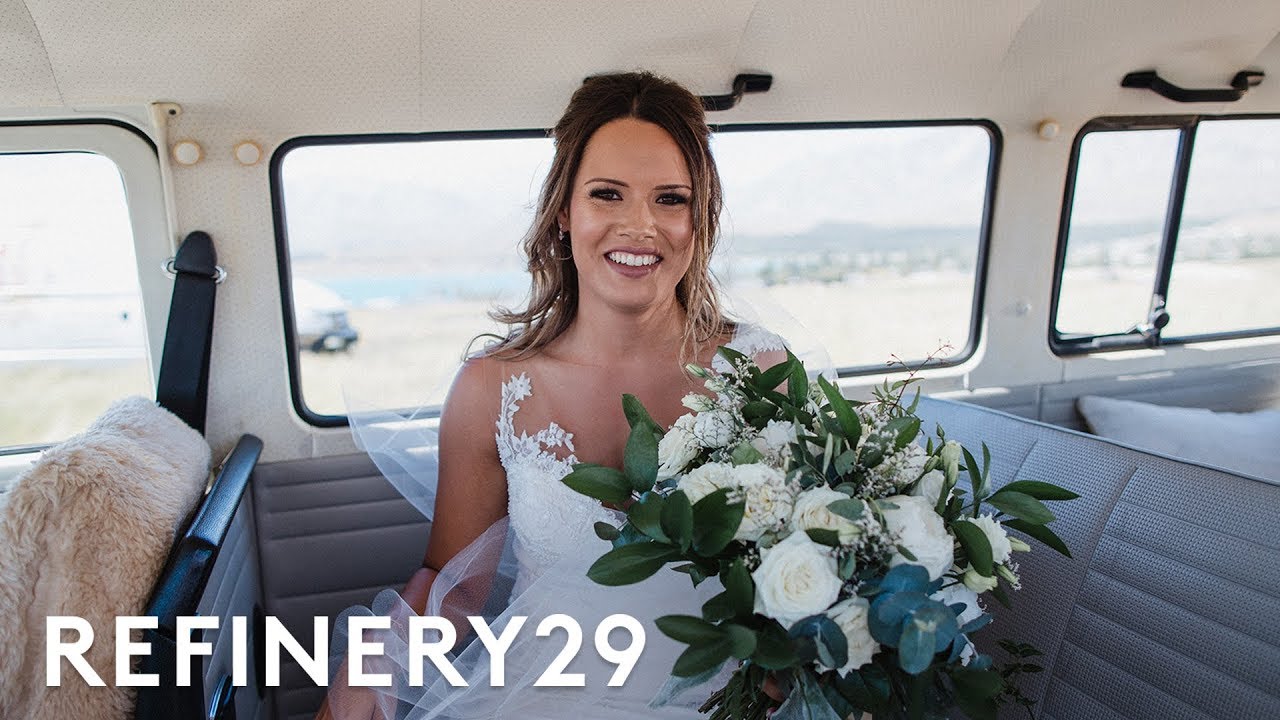In this photograph, we see a woman with dark hair and dark eyes, smiling warmly at the camera. She is dressed in a strapless, white lacy bridal gown, sitting in the middle row of what appears to be a minibus or campervan, indicated by a front seat with a seatbelt next to her and a pillow behind her suggesting a cozy interior. The interior is primarily white with a grayish-silver bench seat visible to her right and a beige-covered seat back to the left. The woman’s hair is pulled back slightly, emphasizing her bright expression. In her hands, she holds a large bouquet featuring mainly white roses, interspersed with a few blue flowers and dark green leaves. Behind her, through the windows, the background is blurred but hints at a bright, sunny day with hills and possibly a beach in the distance. The photo bears the brand name "Refinery 29" at the bottom, framing this intimate moment.